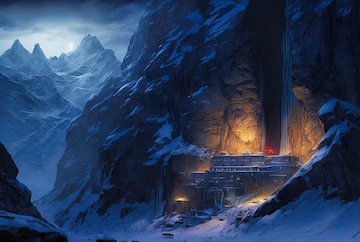The image depicts a striking digital portrayal of an ancient stone fortress nestled within a snowy mountainside, reminiscent of scenes from the Himalayas or the Lord of the Rings. At the bottom center right, glowing lights illuminate the fortress, which is deeply embedded in the mountain, suggesting it serves as an entrance to a cave system. Snow blankets the mountainside and the surrounding peaks, creating a serene yet imposing atmosphere. In the background, behind the central mountain, additional snow-covered peaks extend into the distance, with a dimly glowing moon and clouds hinting at nighttime. The dominant hues of dark blue and gray contrast sharply with the light sources, casting an ethereal glow over the scene and enhancing the fortress's mystical and possibly ancient aura.